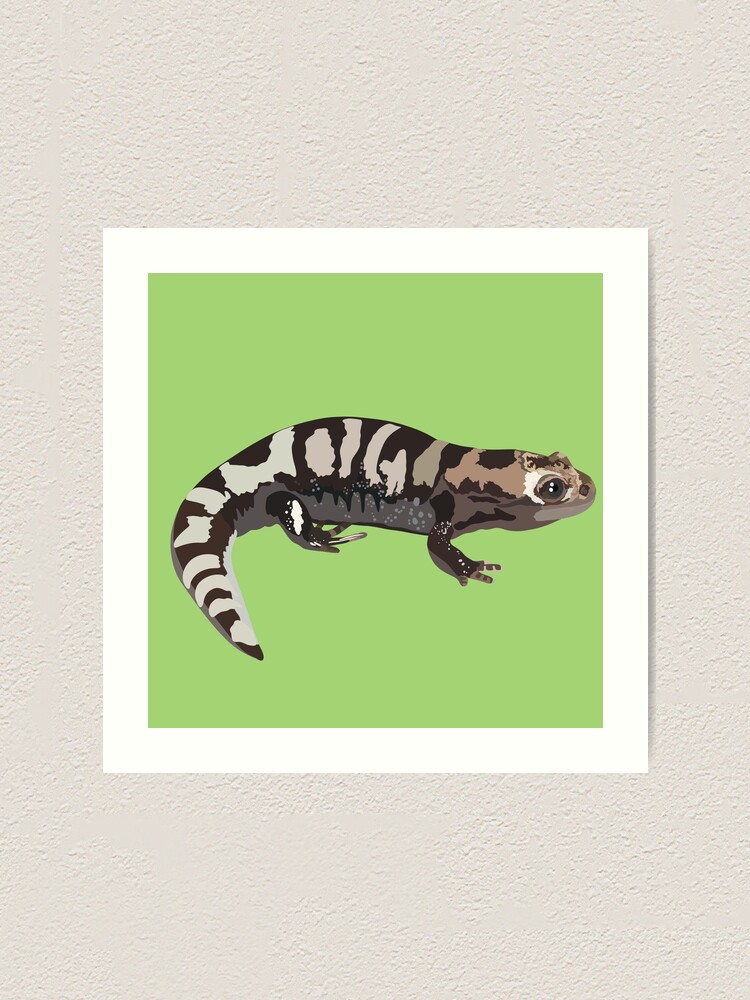The image features a digital art print or painting centered on an off-white, textured wall. The framed artwork has a square format with a white border. Inside the border, the background is a muted lime green, highlighting a central reptilian creature resembling a lizard or salamander. This animal is depicted in a side profile facing left (or right if someone misinterpreted it). The creature showcases a gradient color scheme starting from a light brown head that transitions into a gray tail. Black striping details span across its brown and gray body, with additional white accent stripes especially along the tail. The creature's face bears a frog-like resemblance with prominent black eyes, and it possesses frog-like legs, of which the front and back right legs are visible.